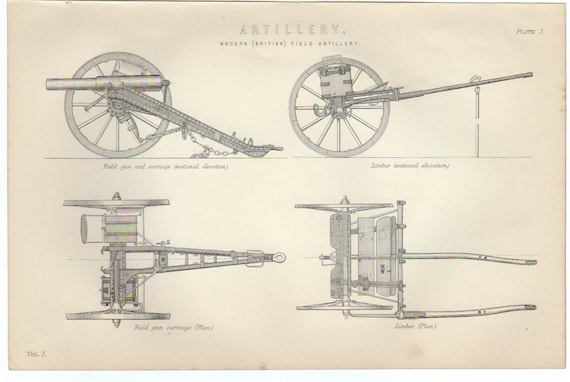The image is a detailed diagram of a modern British field artillery piece, likely sketched in graphite or ink on white paper. At the top of the page, the text "Artillery" is faintly visible, with "Modern British Field Artillery" written underneath in smaller, hard-to-read letters. The diagram features four different views of the artillery, each showing distinct aspects of its structure and components.

In the top-left corner, there's a side profile of the cannon, displaying one of its large spoked wheels and the cannon itself angled towards the ground. Adjacent to this, in the top-right corner, is another side profile where the cannon is angled towards the sky. The two images at the bottom offer top-down perspectives, providing a view of both wheels, the spindle connecting them, and the long arm where the cannon is mounted. The bottom-left view appears to be directly from above, while the bottom-right view could be from below, though it's somewhat ambiguous.

The sketches are annotated with small, barely legible writing beneath each image, offering additional details about the designs. Overall, the diagram provides a comprehensive visual study of the artillery piece from multiple angles.